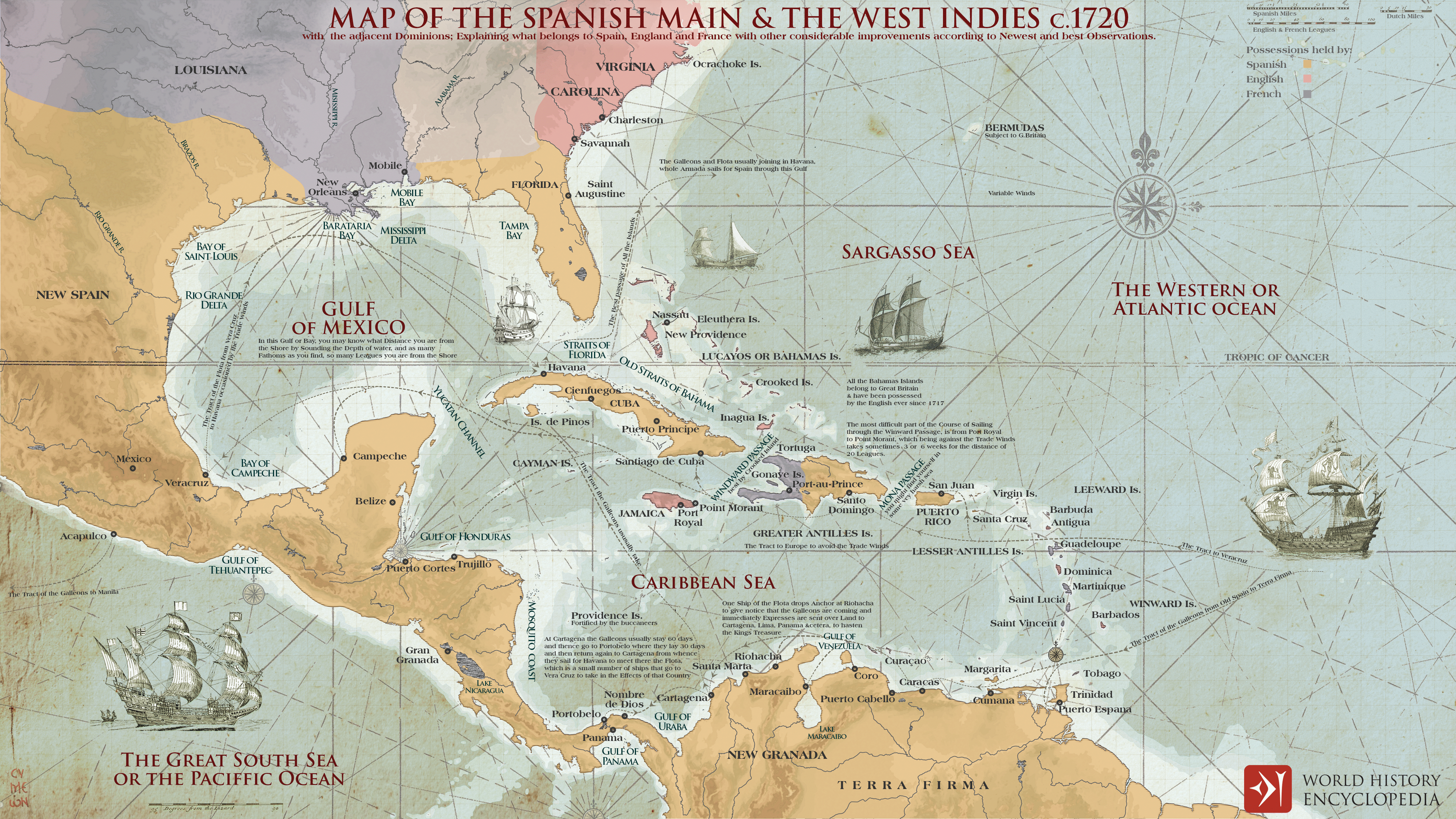This image showcases a modern rendering of a historical map titled **"Map of the Spanish Main and the West Indies, circa 1720."** It provides a detailed view of the southern part of North America, including Louisiana (depicted in purple almost covering the whole region), Virginia, Carolina, and Florida. The map extends to Mexico, labeled as New Spain in yellow, and features parts of South America such as Terra Firma and New Granada. Major bodies of water like the Gulf of Mexico, the Caribbean Sea, the Western or Atlantic Ocean, and the Great South Sea (Pacific Ocean) are marked, with the latter labeled at the lower left. The map is adorned with numerous illustrations of sailships scattered throughout. Color-coding indicates territorial possessions: the Spanish territories are in orange, English in pink, and French in gray, as clarified by a key at the top. Above, the map is annotated in red text with the title and a brief description noting it explains the dominions belonging to Spain, England, and France, emphasizing the newest and best observations of the time. A notable logo in the lower right corner identifies the map's source as the World History Encyclopedia.